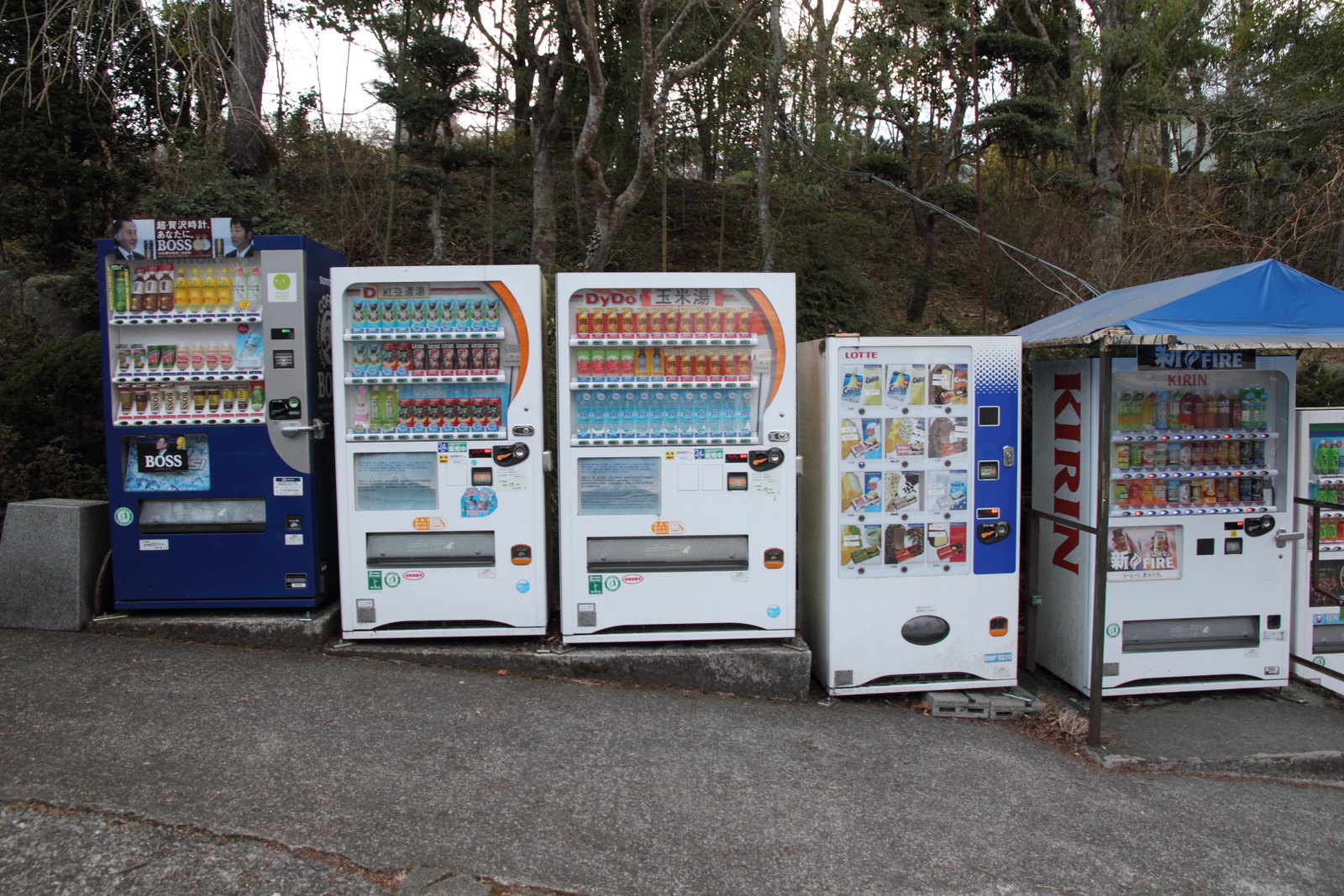The image captures a scenic daytime view of six vending machines arranged in a neat row on a slight downward slope from left to right. The backdrop features a densely packed embankment of green trees with long branches, set against a bluish sky, giving the impression of a park or a serene village setting. In the foreground, there's a noticeable crack on the bottom left of the concrete ground. 

The vending machines vary in color and type. The first one on the left is a distinctive blue machine branded with "Boss," featuring a man's image and a brown label. It offers various bottled drinks. The next three machines are white; the second one contains drinks, the third one labeled "Daido" in the upper left corner also offers beverages, and the fourth, smaller machine appears to sell ice cream or snacks with "Latte" on its upper left corner.

The fifth vending machine stands out with a small blue roof canopy resembling a gazebo, branded with "Kirin" in red writing. It features a variety of beverages, some marked with blue and red lights, which likely indicate availability. The sixth and last machine is partially cut off on the right edge of the image, but you can still see green bottles inside.

Overall, the scene is captured in soft daylight, enhancing the peaceful and somewhat quaint environment.